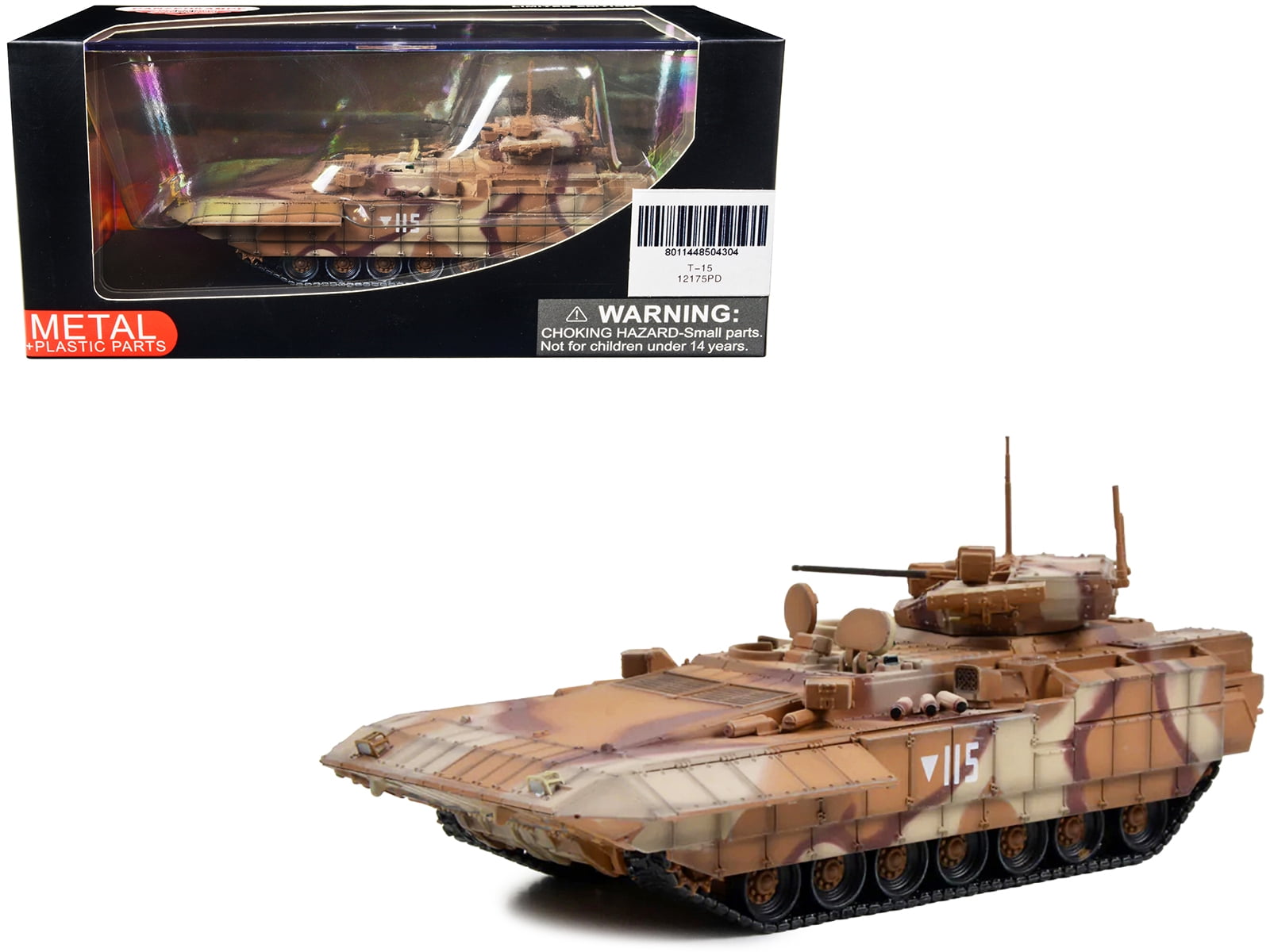The image shows a model of a toy tank in two sections. In the upper left corner, the tank is in its black packaging, featuring a red background with white text that reads "metal and plastic parts." The box also has a barcode labeled T15-12175PD, 801-144-8504-304, and a gray warning label stating, "Warning: choking hazard, small parts, not for children under 14 years." The packaging has a plastic see-through window allowing a view of the tank inside. 

The tank itself, prominently displayed out of the box in the bottom right section of the image, boasts a detailed design with camouflage colors in shades of dark brown, light brown, and off-white. It features black treads, a rotating turret on top, various antennas, and radar equipment. The number 115 is printed on the side of the tank, accompanied by a downward-pointing arrow. The tank's colors suggest a desert military theme, enhancing its camouflage effect. This comprehensive view of the model highlights the intricate details and craftsmanship of the toy tank as it would appear both on display and taken out of the packaging.